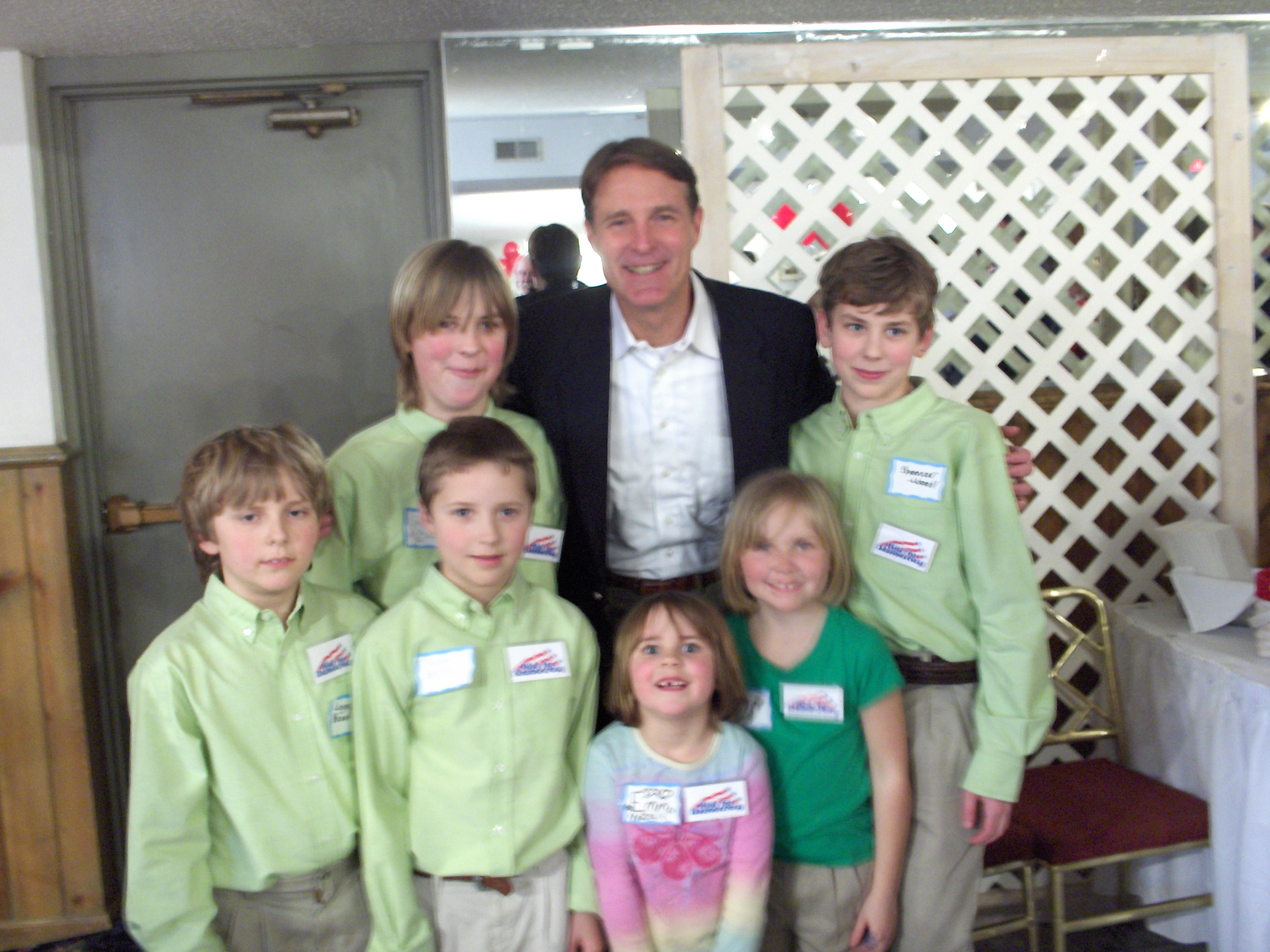A group of seven people, comprising a man and six children, poses for a photograph in a room that might be a restaurant. The man, positioned centrally behind the children, is attired in a suit jacket over a collared, button-down white shirt. He has his arms gently placed around two boys, each standing to his side. All four boys in the image are wearing light green, long-sleeve button-down shirts adorned with two name tags. One tag seems to feature text and a red design, although the details are indistinct.

In front of the boys, two girls are positioned at the front and are visibly smiling along with the rest of the group. One girl is dressed in a green t-shirt while the other wears a pastel-colored, long-sleeve shirt. The background reveals a white lattice wood panel on the right side and a gray door on the left, which appears to lead outside. The lower right corner of the image showcases a red chair with a gold back, adjacent to a table covered with a white tablecloth.